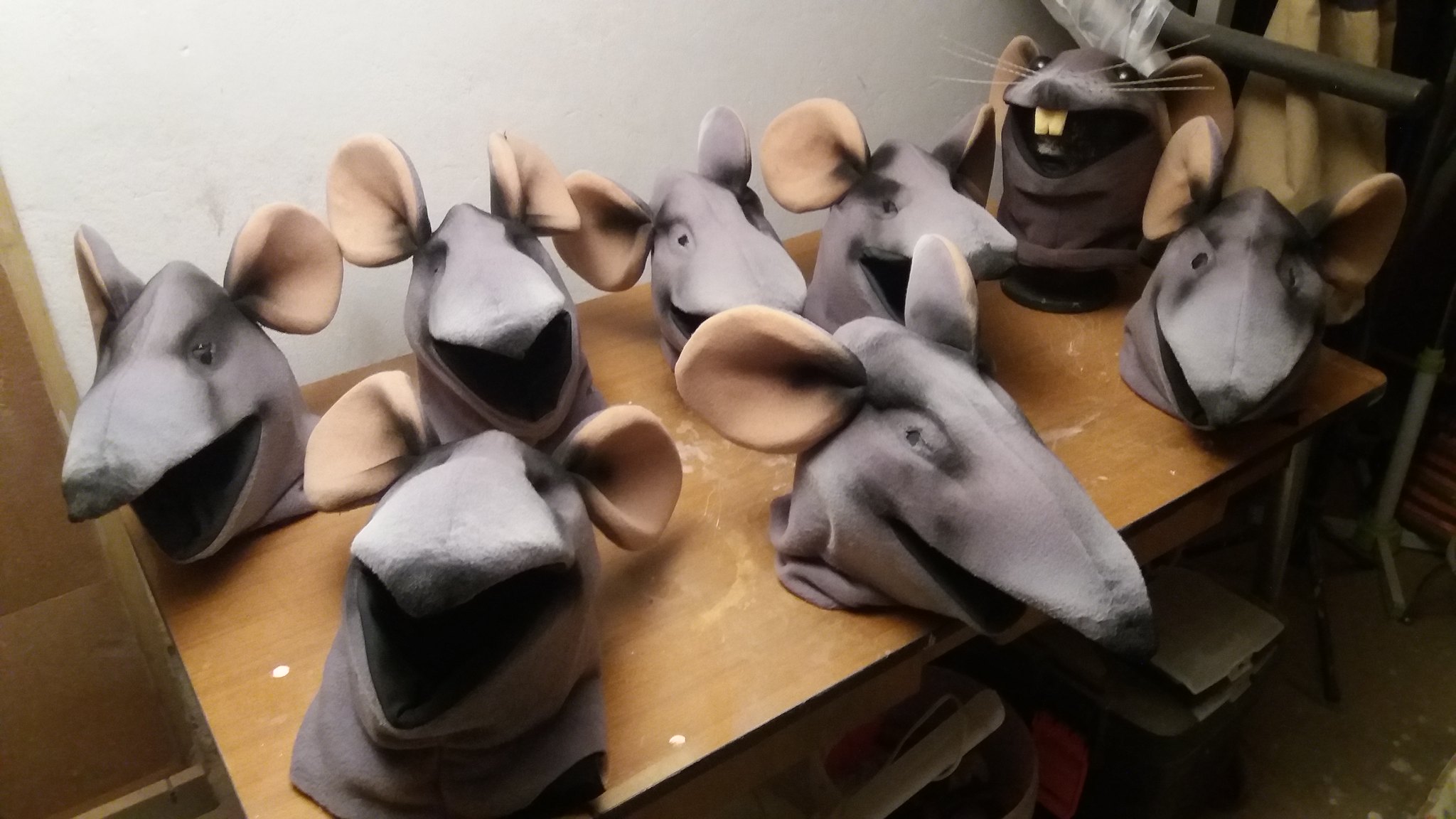This color photograph captures a quirky scene of eight rat head puppets arranged on an old wooden desk, which shows signs of wear with chipped paint on the surface. Each puppet, designed to be operated by hand, has a gray face with long noses and tan ears. Most of these rodent characters are incomplete, lacking eyes, teeth, and whiskers, except for one notably detailed puppet positioned at the back right. This specific rat head has glassy eyes, protruding whiskers, and an open mouth revealing two sharp front incisors. Tucked beneath the desk are some stools, and the background is a simple white or partition wall. The setting gives off an educational or creative arts vibe, possibly within a school's theater department, with the feet of a music stand or similar object visible in the background.